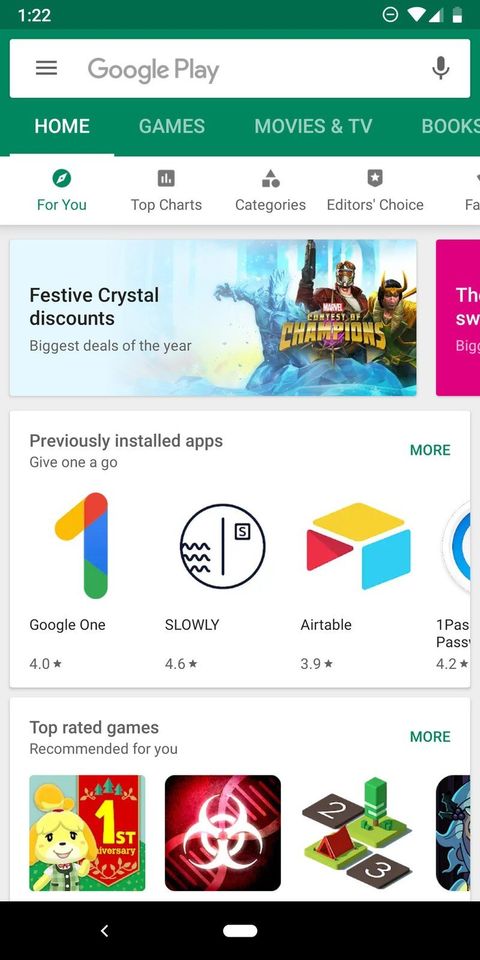A screenshot of a smartphone display demonstrating a Google Play Store interface. At the very top, a green notification banner displays in white text "12:22" (with ambiguity whether it's AM or PM), followed by indicators showing a strong internet connection and approximately 50% battery life. Below the green banner is the main Google Play Store header. On the left, there is a hamburger menu icon, with a microphone icon to the right of it. 

The green header bar contains navigation options: "Home" is highlighted in white, indicating the current section. To the right are other categories in white text: "Games," "Movies & TV," and "Books." Beneath this header is a white background section with several tabs: "For You" is selected, showing personalized content. Other available tabs are "Top Charts," "Categories," "Editor's Choice," and an off-screen option.

In the "For You" section, featured items include:
- "Festive Crystal Discounts," likely a promotional event or game-related discount.
- A game from Marvel, possibly "Contest of Champions."
- A section titled "Biggest Deals of the Year," partially obscured and highlighted in pink.

Further down, a section titled "Previously Installed Apps" offers suggestions. Visible apps include:
- Google One, rated 4.0 stars.
- Slowly, rated 4.6 stars.
- Airtable, rated 3.9 stars.
- Another app rated 4.2 stars, partially cut off.

A green link labeled "More" allows additional exploration of this section. Below this, a list of "Top Rated Games" is available for selection.